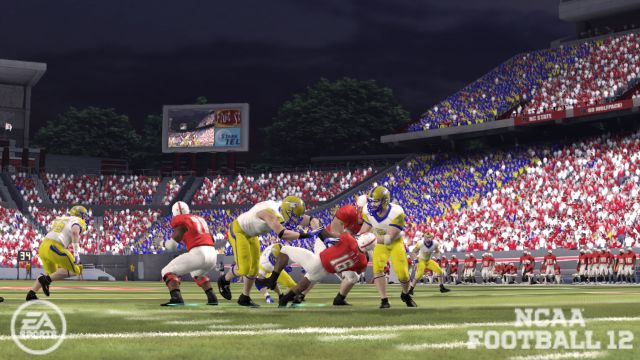The image depicts a dynamic scene from a football video game, likely played on a computer or gaming console. The grandstands on the right side of the field are densely packed with vibrant crowds, adorned in a mix of red and white, and royal blue colors, creating a vivid tapestry of fan sections. Although individual spectators aren’t clearly visible, their collective presence is implied through the colorful mass. 

The aisles divide these sections distinctly, with the central upper stands showcasing a prominent red and white section, bordered by blue-clad fans in front and more red and white supporters towards the back and left. Adjacent to the stadium, lush green trees form the backdrop, adding a touch of natural scenery.

The football field itself is grass, and the game is in full swing. Players in red and white uniforms, featuring red tops with white numbers, white helmets with a red stripe, white pants, and red socks, face off against an opposing team in white shirts, yellow helmets with blue stripes, yellow pants with blue stripes. 

On the right side of the image, high above the grandstands, a large screen is visible, with trees peeking behind it. In the top right corner of the screen, the text "NCAA Football 12" is prominently displayed, while the top left features a round white circle with the "EA Sports" logo, suggesting this is likely a scene from the popular NCAA Football 12 video game.